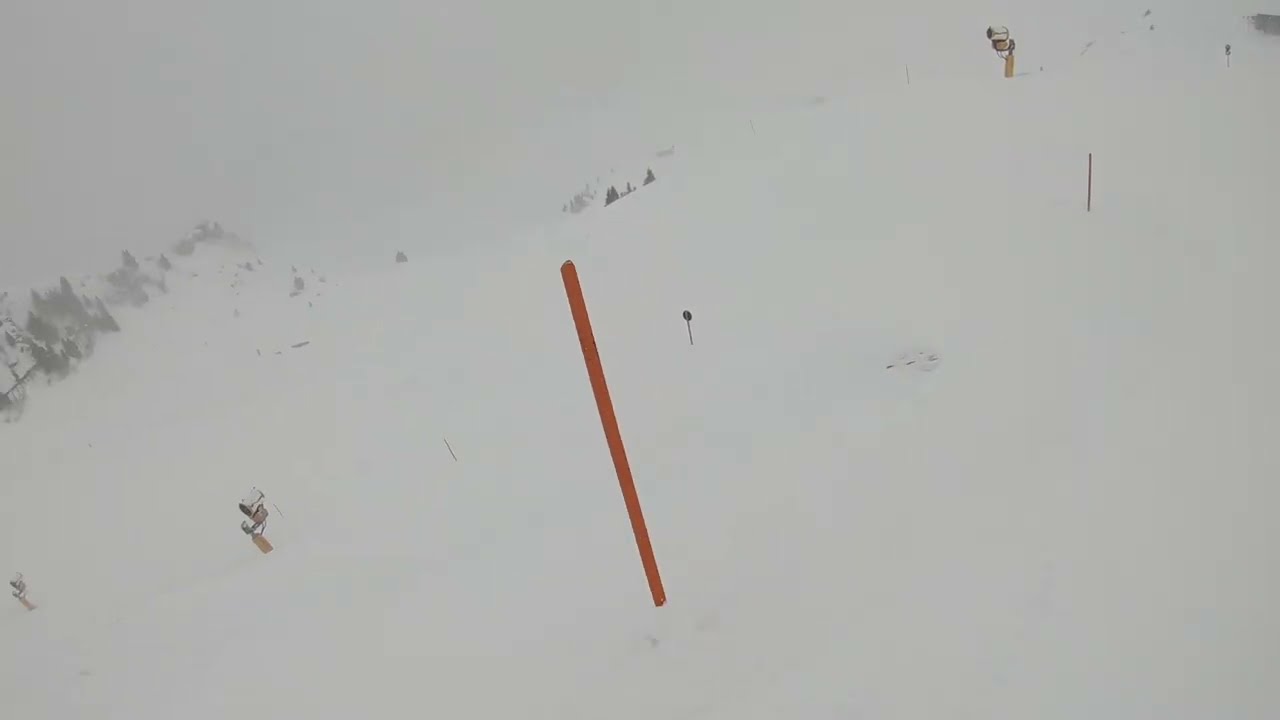This is a horizontally aligned rectangular picture of a snowy landscape, dominated by fresh, untouched snow. The scene depicts a wintry day on a snow-covered mountaintop, enveloped in a grayish-white sky with no visible sun or clear blue sky. In the very center of the image stands a thin red (possibly orange) pole, likely used for measuring snow depth or marking trails, slightly angled. The snow appears smooth and pristine, with a single visible footprint near the red pole.

On the far left side of the image, green trees rise through the snow, adding a touch of color and indicating the presence of a hill or slope behind them. In the center background, there appears to be another object that resembles a mailbox, barely visible and poking through the snow, possibly serving as a boundary marker.

In the upper right-hand side of the picture, there is a shorter, brown pole sticking out of the snow. Some other indistinct, black dotted features dotting the background might be additional trees or other landscape elements, though they are difficult to precisely identify. The serene, untouched snowfield encapsulates the cold, tranquil ambiance of this winter scene.